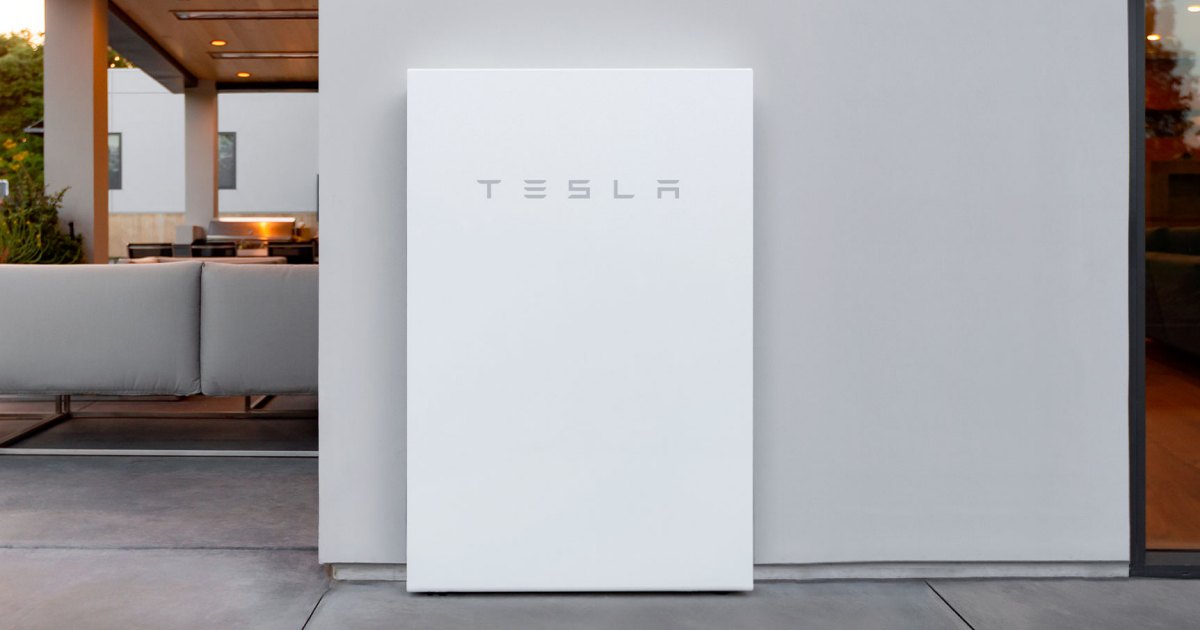This photograph captures a section of an outdoor, yet covered, patio area likely associated with a Tesla facility. The setting features a wooden ceiling adorned with downlights, creating a warm, inviting atmosphere. The space is architecturally unique, with large open window frames bordered by structural support beams, allowing an abundance of natural light to flood in. 

Under the ceiling, elegant light gray leather seating and neatly arranged tables provide a modern, comfortable feel. The seating area extends across a large, gray tiled sidewalk, adding to the sleek, contemporary design. In the background, some neatly maintained bushes add a touch of greenery to the otherwise industrial aesthetic.

Against a gray wall, which is about two to three feet high, leans a lighter gray rectangle. At the top of this rectangle, the Tesla emblem and wordmark stand out in a slightly darker gray, subtly promoting the brand. To the right of this wall, a black-framed window offers a glimpse into the interior of the building, revealing a continuation of the sleek interior decorated with wood flooring.

Overall, this image highlights a blend of modern architectural elements and sleek design, reflecting the innovative and upscale brand image of Tesla.